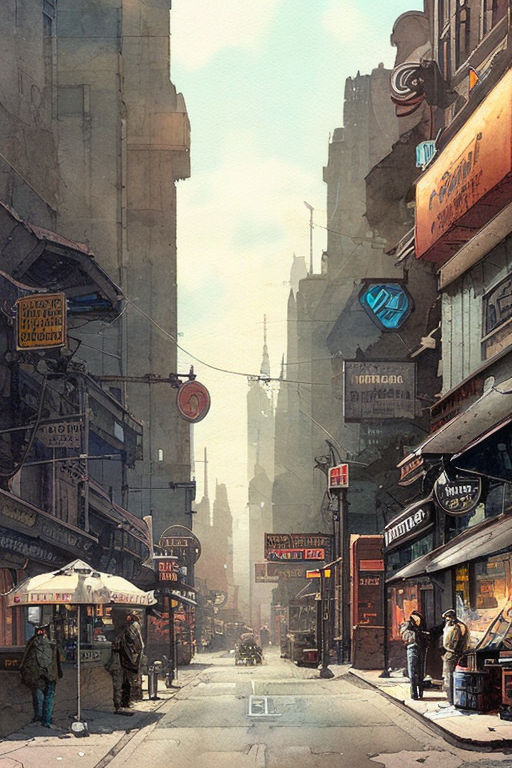A detailed painting of an old, industrialized urban street scene, possibly set in an Asian city from about 70 to 80 years ago. The colors are predominantly gray and brown with sporadic splashes of color, such as reds and whites that punctuate the scene. The atmosphere is somewhat bleak and hazy, contributing to a foggy ambiance. The street, lined with tall buildings that range from multiple stories to potentially as high as 70 or 80 stories, extends into the distance where spires, possibly from churches, are faintly visible.

The foreground features a road, possibly housing an old car or a horse-drawn carriage. Sidewalks on both sides are populated with people chatting and walking, lending a sense of life to the scene. To the left, there's an umbrella shading a retail storefront, characteristic of old-time businesses with awnings and protruding signs on poles. On the right, there appears to be a newsstand with a vendor leaning against it. None of the signs or advertisements are in English, enhancing the foreign and nostalgic feel of the setting. The overall scene, while a bit rundown and 'rust-belty,' evokes a quaint, historical charm rather than an unsafe atmosphere.